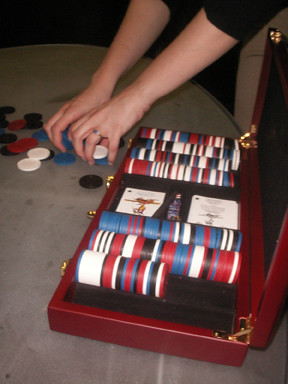This image captures a detailed scene of a poker chip case, which is positioned open on an oval, tannish-gray table. The case, crafted from reddish wood and fitted with gold latches, features a black interior with felt slots for the chips. Inside the case, there are organized rows of poker chips in black, red, white, and blue; the back holds four full stacks, while the front has two full stacks, one half-empty slot, and one completely empty slot. Centrally located are spaces likely meant for playing cards, with a couple of white cards visible. A person with a black, elbow-length sleeve shirt and a silver wedding ring is reaching into the case with two hands, presumably to place the remaining chips from the table into the empty slots. The setting suggests that the game has concluded, and the chips are being neatly stored away.